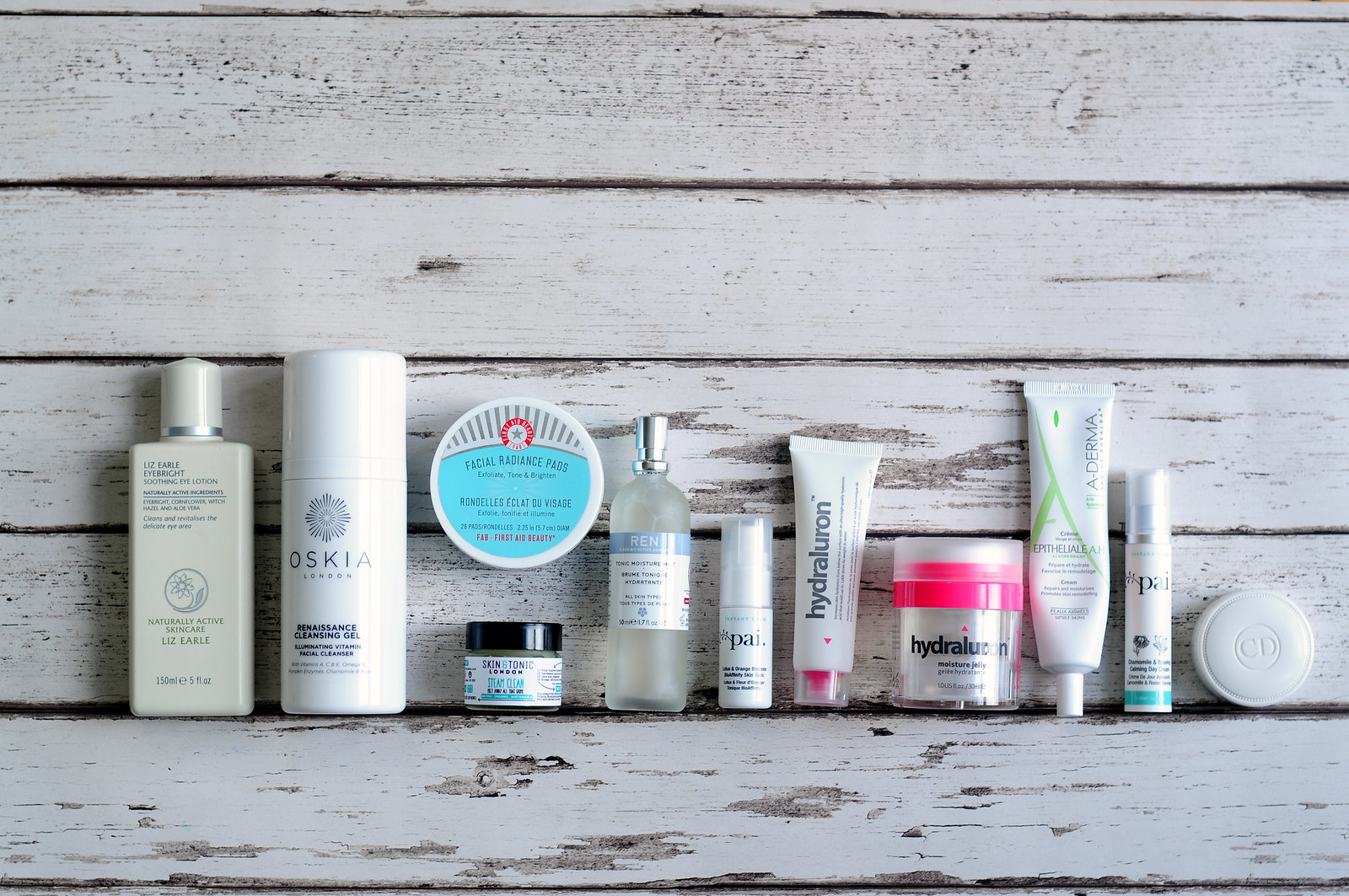The color photograph showcases a neatly arranged collection of beauty items on a clean white wooden surface. Each product, meticulously placed from left to right, reflects a diverse array of skincare essentials.

On the far left, a square bottle with a white cap prominently displays its brand, "Liz Earle," and is labeled "Eye Bright Soothing Eye Lotion." The detailed text highlights its naturally active ingredients including cornflower, witch hazel, and aloe vera, intended to clean and revitalize the delicate eye area. The label also features a floral emblem within a circle and notes the product volume as 150 milliliters (5 fluid ounces).

Adjacent to Liz Earle, there is a round white bottle with a starburst design on the top of the label. The text reads "OSKIA London, Renaissance Cleansing Gel," touting it as an illuminating vitamin facial cleanser.

Further along, at the top of the layout, sits a round container with a blue and silver label. It is identified as "Facial Radiance Pads" from "First Aid Beauty," detailing its purpose to exfoliate, tone, and brighten with a count of 28 pads measuring 2.25 inches in diameter.

Below this container lies a small pot with a black lid, labeled "Skin & Tonic London, Steam Clean," though the rest of the text is not readable.

To the right, a clear frosted glass bottle capped with silver is labeled "REN Tonic Moisture." Next in line is a small white bottle with a clear plastic cap, marked "PAI," though the writing is too blurry for further details.

A white tube follows, identified as "HYDRALURON" with a clear plastic cap revealing a pink nozzle inside. Adjacent to this, a pot also labeled "HYDRALURON Moisture Jelly" features a frosted top with a striking hot pink edge.

Following these, there's a tall white tube marked "ADERMA," distinguished by a green diagonal line, though the label is too blurry to read fully. Next to it stands another small white tube labeled "PAI."

Finally, the collection concludes with a circular product marked with "CD" at the center, suggesting it is a product by Christian Dior.

The organized ensemble of skincare items highlights an impressive variety of brands and products, designed to cater to diverse beauty needs.